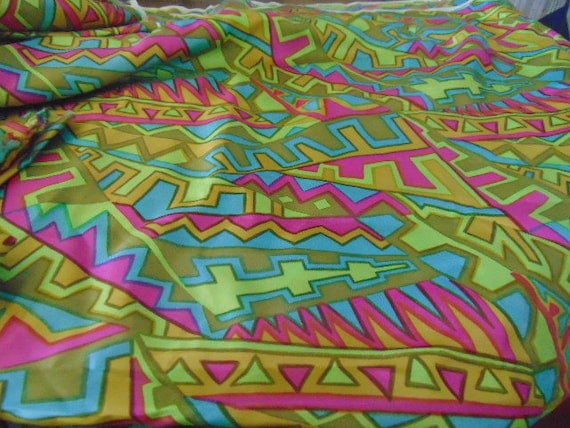The image depicts a vibrant and colorful piece of fabric, likely a blanket or bedspread, displayed in a close-up view that highlights its intricate details. The dominant background color is a light, sky blue, interspersed with geometric shapes including squares, arrows, and triangles, all rendered in vivid shades of pink, green, yellow, and gold. The patterns exhibit an eclectic, almost 70s-inspired design featuring light green and dark green shapes, with some dark green outlines. Among the most striking elements are tall, pink zigzag lines resembling a child’s representation of mountains, enhancing the fabric's dynamic and lively appearance. The overall clarity of the image is high, allowing one to appreciate the bright and clear setting, free from any textual or numerical distractions.